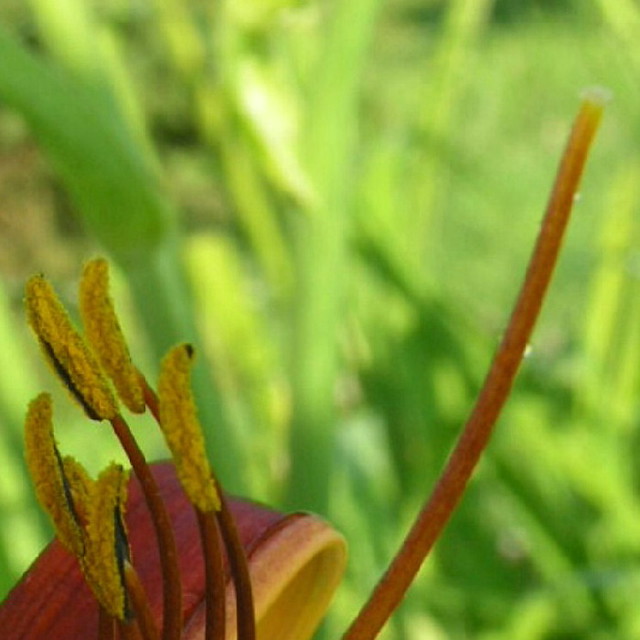This low-resolution, blurry photograph captures a scene dominated by vibrant plant life, set against a sunlit background of varied green leaves. Central to the image is a striking red leaf with a yellow-edged, curled appearance. In front of this red leaf are several delicate filaments: they have brown stalks and extend into long, narrow tips touched with bright yellow, particularly abundant in the bottom left area of the picture. Notably, on the right side, there's a prominent filament with a long, brown stem but lacking the yellow tip seen on others. The overall background scene includes a mix of brighter and lighter green leaves, contributing to the sun-drenched setting of the photograph.